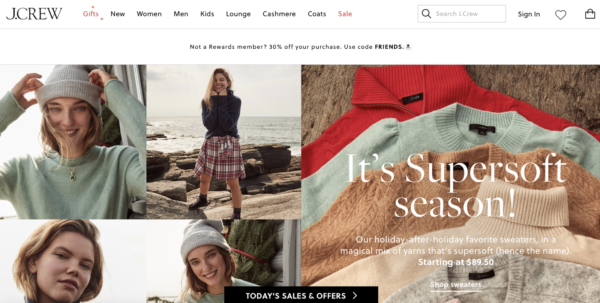This is a screenshot from a shopping website with a white background. In the top left corner, "J.Crew" is displayed. To the right, there's a horizontal menu with options labeled "Gifts," "New," "Women," "Men," "Kids," "Lounge," "Cashmere," "Coats," and "Sale." A search bar with a black magnifying glass icon is positioned beside the menu. Further to the right, it reads "Sign In" followed by icons: a heart and a shopping bag.

Below the menu, a white promo bar appears with text that reads, "Not a rewards member? 30% off your purchases. Use code FRIENDS." 

The main section of the screenshot features several images. On the left, a white, blonde woman is standing on a rocky beach, dressed in a heather gray sweater, a necklace, and a beanie. Next to her, another white, blonde woman also stands on the beach, wearing a black sweater and a plaid skirt reminiscent of a Catholic school uniform. To the right, there is a neatly stacked pile of sweaters in colors: red, gray, brown, beige, and another gray. Overlaid on the sweaters in white font are the words, "It's super soft season."